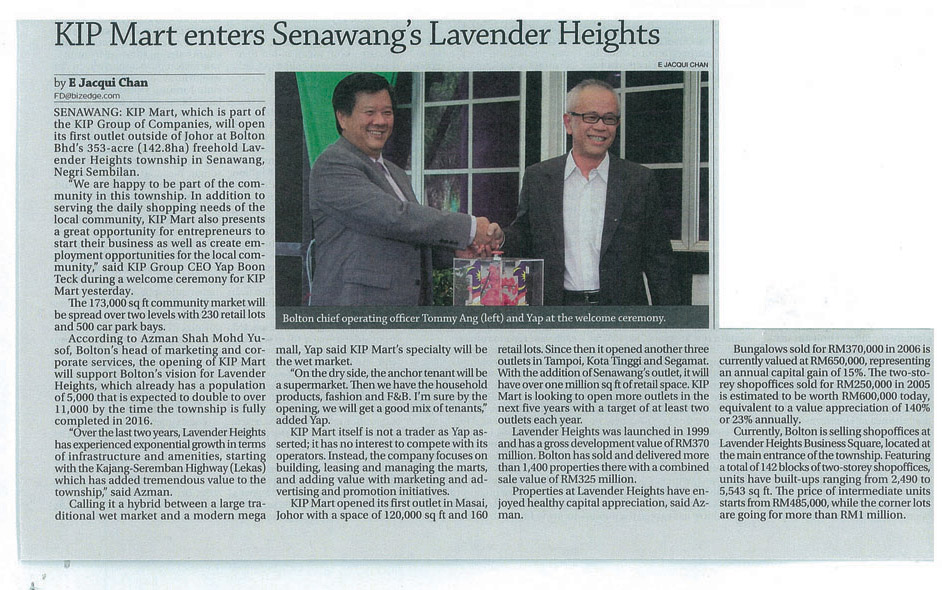This is a rectangular newspaper clipping with a missing section on the right side, giving it a slightly irregular shape. Dominating the upper-center of the clipping is a photograph featuring two men in suits, smiling and shaking hands. The man on the left, with black hair, is Tommy Ong, the Chief Operating Officer of Bolton. The man on the right has gray hair and is identified by the caption as participating in the welcome ceremony. Both men have Asian features. The title of the newspaper clipping reads, "KIP Martin Enters Santa Wings, Lavender Heights." Surrounding the photograph is an article authored by Jackwee Chan, detailing the opening of a new KIP Martin location in the Lavender Heights township of Santa Wong. The unusual cut-out section on the right seems to be an attempt to include the entire length of the article in the clipping.